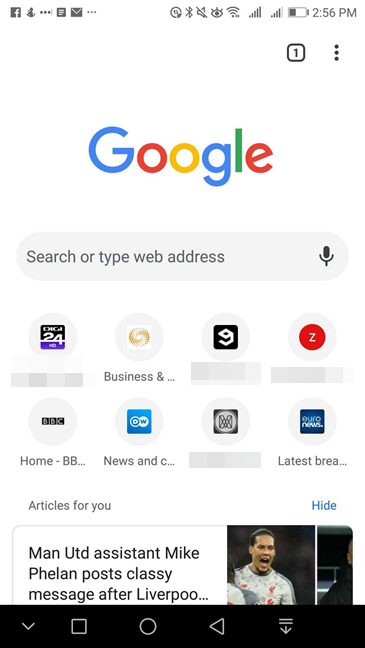This image is a detailed screenshot of a smartphone display, currently on the Google homepage. 

At the very top left corner, there are several gray icons, including a recognizable Facebook icon among others that are not identified. Next to them, moving right, there's a Bluetooth icon, a muted speaker icon, an eye symbol, a Wi-Fi icon, and signal bars indicating cellular service strength. Further to the right, the battery indicator shows it is below 50 percent charged, and the time is 2:56 p.m. Below the battery icon, a notification shows a black number "1" inside a small black square with a white interior, flanked by three vertical dots to its right.

Dominating the center of the page is the Google logo against a white background. Directly beneath it is the search bar with the prompt "Search or type web address," accompanied by a speakerphone icon on the right end of the bar. 

Below the search bar are several app icons. One is black, white, and purple labeled "24". Another is a gold swirling circle, followed by a partially visible white cube icon, and then a red circle with a white "Z" in it. Underneath the gold swirling circle, the text reads "businesses..." 

Beneath these icons, various news outlet logos are visible, including the BBC, DW, and RONews. Additional labeled sections beneath the logos read "home", "BBC", "news", and additional text that trails off with "...see." 

At the very bottom, there is a news headline reading, "Man UTD assistant might fill on post classy message after Liverpool," accompanied by a picture of an athlete. Finally, the navigation buttons are clearly present at the bottom of the image in black.